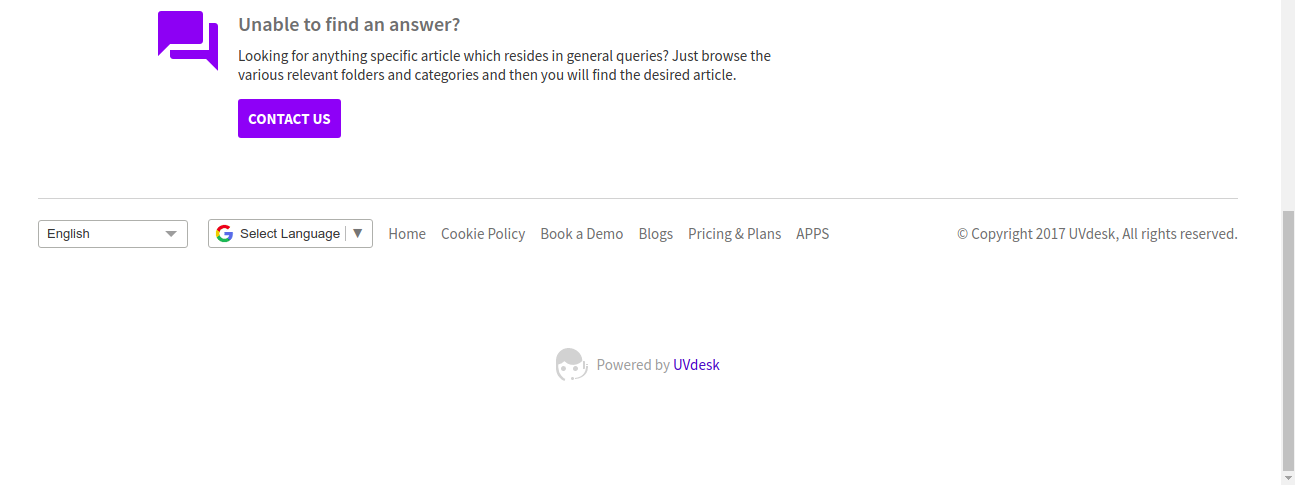This is a detailed description of a screenshot in landscape mode, with a predominantly white background. The image is divided into two rows, featuring a scroll bar on the far right side, positioned at the bottom half. 

In the upper row, towards the left-center, there's a message stating, "Unable to find an answer? Looking for a specific article? Browse the various relevant folders and categories, and then you will find the desired article." Below this message, a purple button reads "Contact Us," and to its left is a purple and white logo resembling a messaging icon.

In the lower row, the content begins with a drop-down menu for language selection, showing "English." Next to it is another drop-down menu with the Google logo, labelled "Select Language." Following these menus are category headers, which include "Home," "Cookie Policy," "Book a Demo," "Blogs," "Pricing and Plans," and "APPS." 

To the far right, the text reads "Copyright 2017, UVdesk, All rights reserved." At the very bottom, there is a live link stating, "Powered by UVdesk."